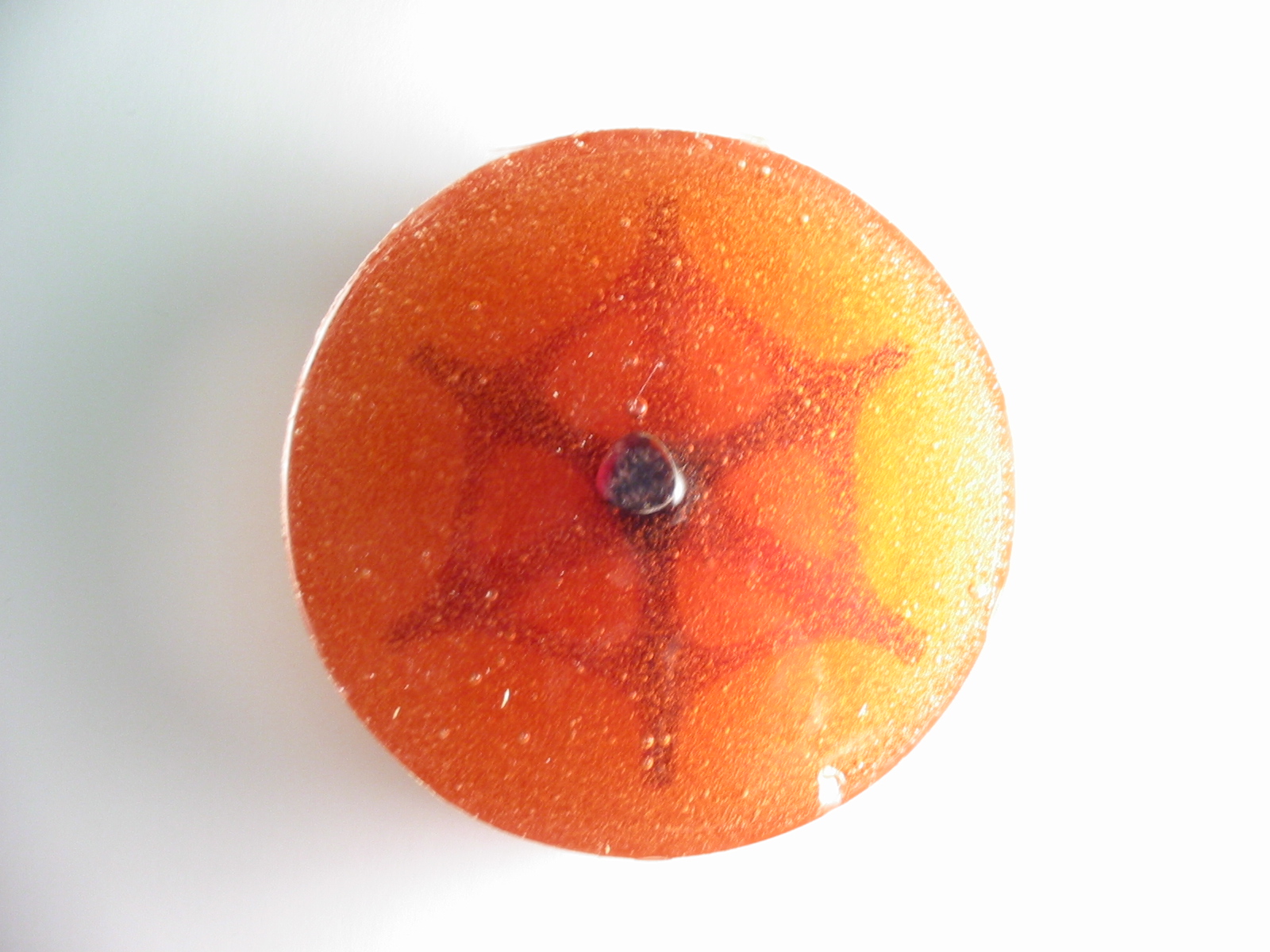This photograph showcases a circular object that is predominantly orange, with a gradient that fades to a lemony yellow on the right side. The surface of the circle is adorned with tiny flecks of white. At the very center, there is a metallic, silver circle that runs through it, appearing to anchor the structure. The object, which resembles a plastic or polymer wheel, is semi-transparent, revealing a reddish-orange star-like design within it. This internal design has six points and six lines that radiate from the central silver circle, reminiscent of an old ship's steering wheel. The wheel is placed on a white surface, and the lighting is brighter on the right side of the image, casting a slight shadow on the left, indicating the light source is to the right. The background and the circle itself are also slightly darker on the left side.